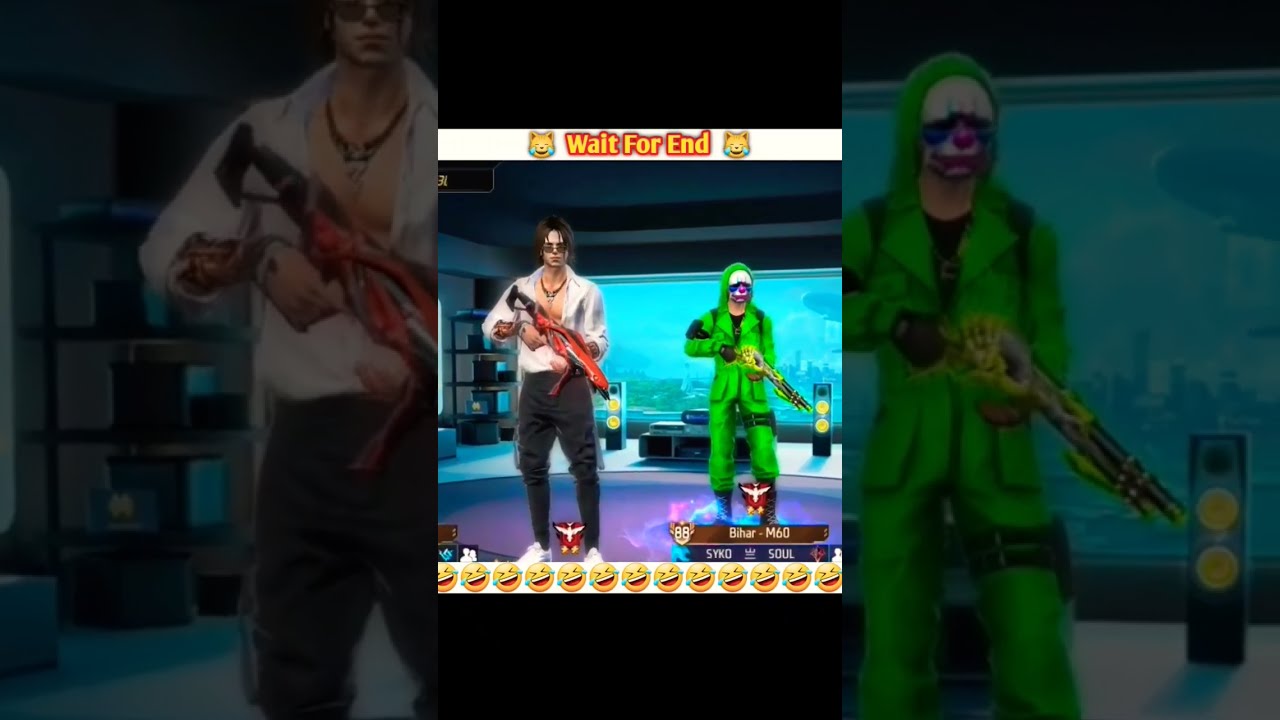The image appears to be a screenshot from a video game set in a room with a blue background. In the center, there are two characters standing on a round, purple surface. The character on the left is dressed in a white coat or shirt that is open at the chest, paired with black pants and sunglasses, wielding a large red gun. The character on the right is dressed in a green outfit resembling an army tracksuit with boots and a clown mask, holding a yellow and green gun. Behind them, the background includes a darkened and zoomed-in version of the same image with what seems to be a large window and a bookshelf with speakers.

At the top of the image, text reads "wait for the end" in orange, accompanied by two cat emojis that appear to be smiling and crying. Along the bottom edge of the screen, there is a line of crying-laughing emojis. Additionally, there are unreadable lines of text on the bottom right corner, identified as "BRM60" and "SYKDSOUL."